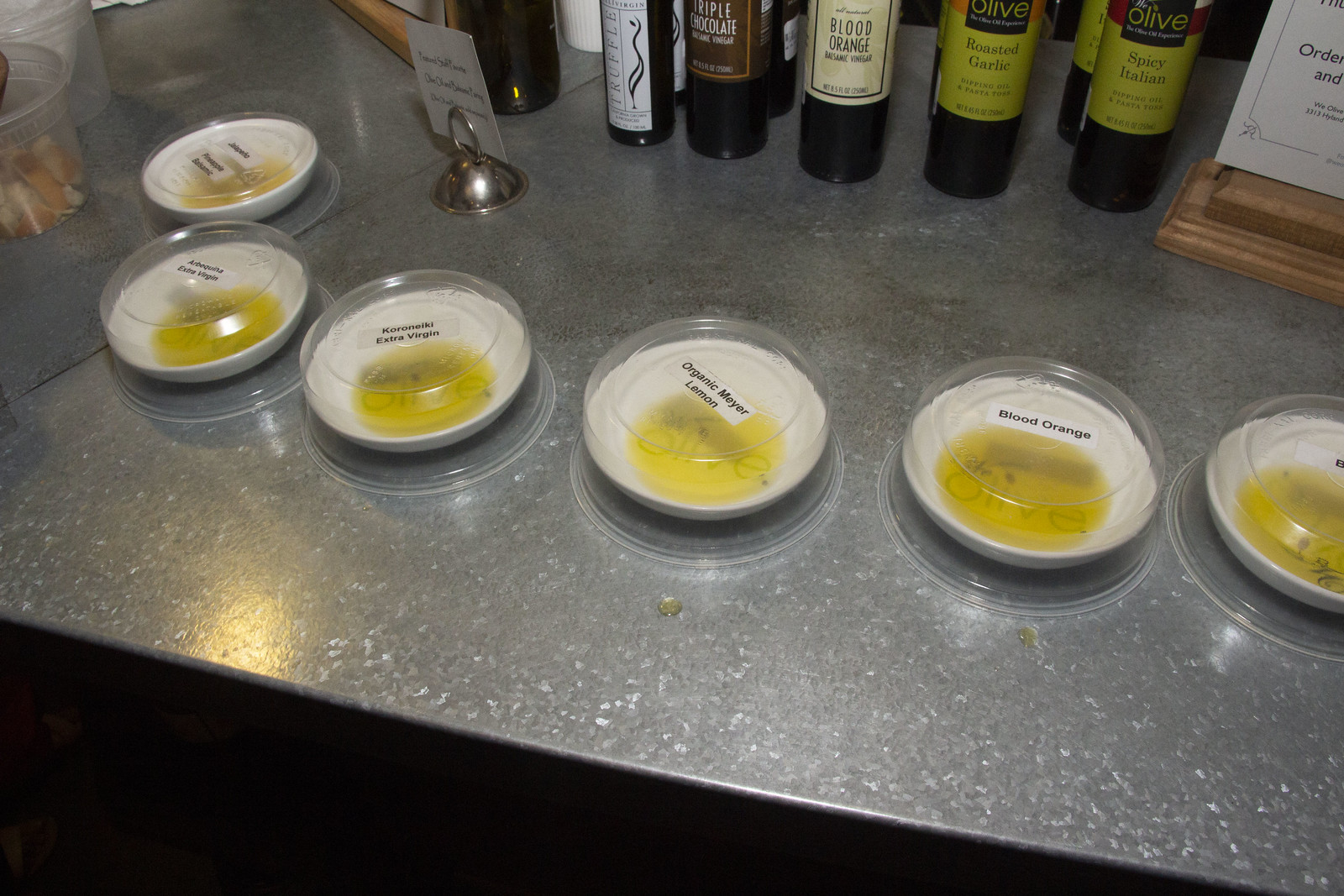The image depicts a gray granite countertop adorned with several clear plastic containers, each with a labeled lid. The labels on the lids feature white backgrounds with black fonts, including descriptions like "Organic Meyer Lemon" and "Blood Orange". These containers appear to hold flavored olive oils. Positioned behind them is a row of bottles, possibly additional varieties of flavored olive oils, with labels like "Roasted Garlic," "Spicy Italian," and "Blood Orange". To the right of the scene is a small wooden stand holding a piece of paper, and to the left is a circular metal stand also displaying a piece of paper. The setup seems to suggest an olive oil tasting.